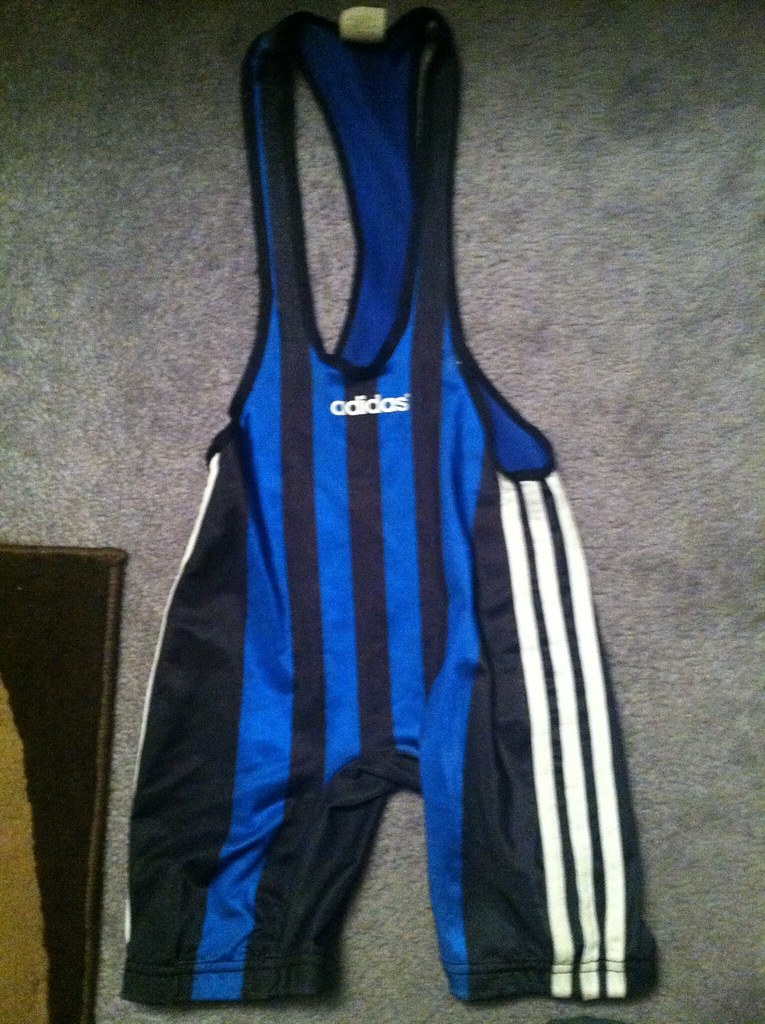This detailed photograph captures a sportswear garment, reminiscent of a wrestling singlet or possibly a cyclist's outfit. The Adidas-branded one-piece is designed with a hole for the head, two armholes, and two leg holes, indicating it's a sleeveless jersey with integrated shorts. Made from elastic, spandex-like material, the singlet features royal blue and black stripes running vertically along the body, while the legs are adorned with white vertical stripes against a contrasting background. The front of the garment prominently displays the Adidas logo in white text beneath the head hole. The sleek outfit is laid out flat on a gray carpet, with a corner of a decorative picture frame or mat featuring golden and black detailing visible in the image.